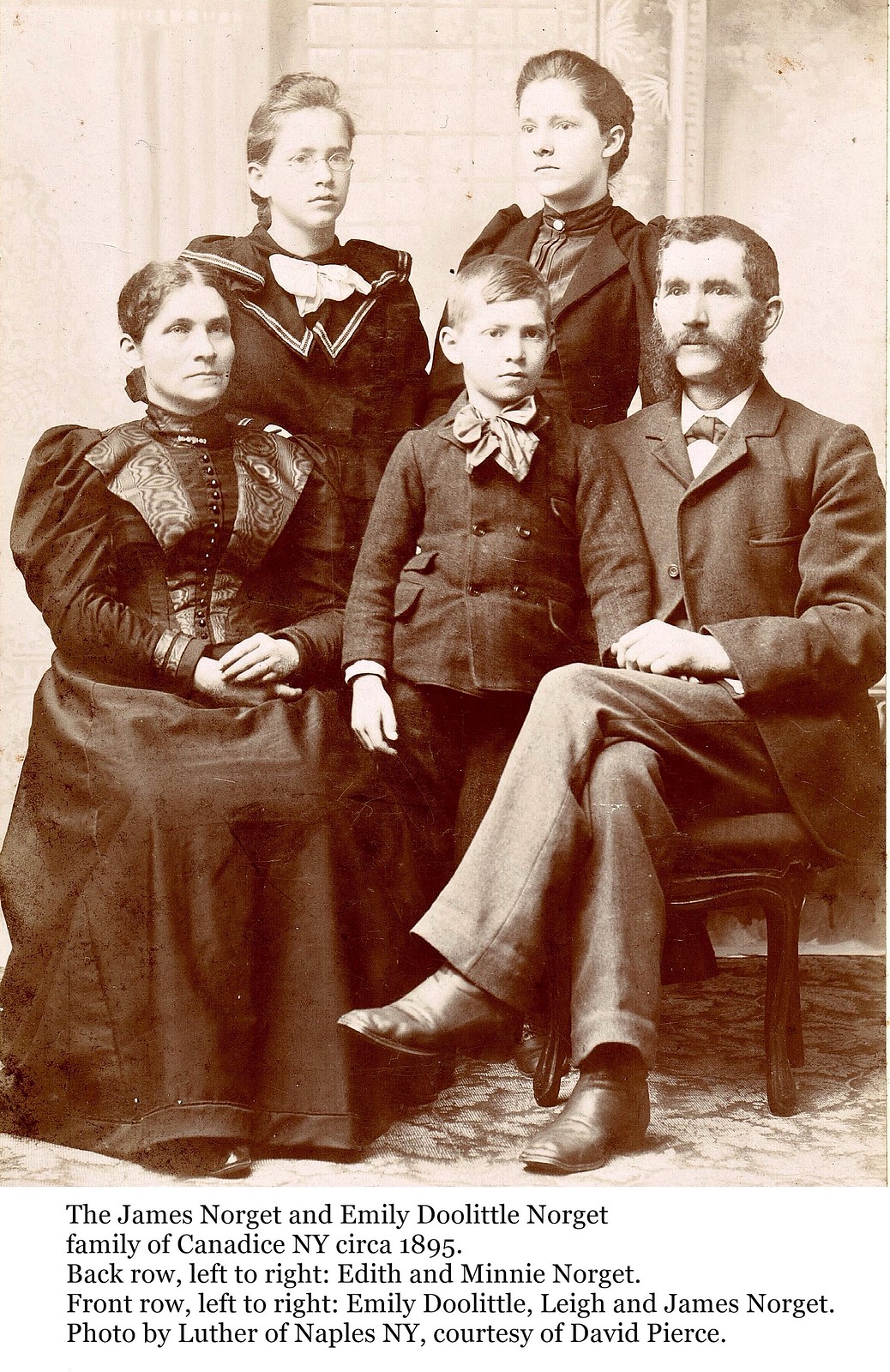The sepia-toned photograph, dating circa 1895, depicts the James Norgat and Emily Doolittle Norgat family of Candace, New York. It shows five family members dressed in formal, conservative attire reminiscent of puritanical style. Seated on the left, Emily Doolittle Norgat is captured with a stern 'stork-like' appearance, while James Norgat, on the right, dons an Abe Lincoln-esque suit. Between them sits a young boy, presumably their son, who is flanked by his two older sisters standing behind; the daughters are identified as Edith and Minnie Norgat. The black text at the bottom provides further details, noting that the photo was taken by Luther of Naples, NY, and is courtesy of David Pierce.